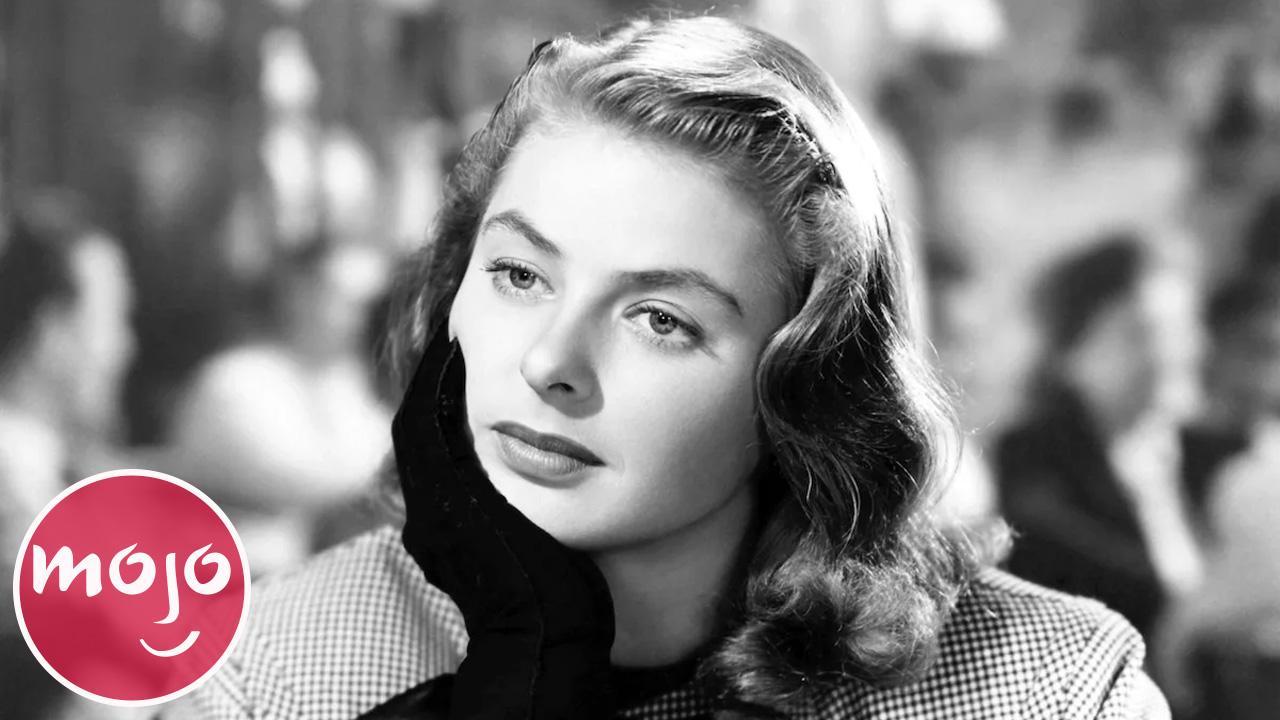This black and white photograph captures a contemplative scene with an older cinematic style, likely from the 40s or 50s. The image centers on a striking woman, possibly a famous actress, seated and resting her chin on a gloved hand. She exudes a pensive elegance with her wavy, shoulder-length blonde or light brown hair, which is parted to the side. Dressed in a jacket featuring a small checkered pattern, she gazes intently to the left, her eyes suggesting deep thought or attentive listening. 

Positioned in the lower left corner is a distinctive red logo for "Mojo." The logo is a creative design with the letters M-O-J-O arranged to form a smiley face, accentuated with white letters. The surrounding environment is blurred but implies a lively restaurant setting, with indistinct figures mingling in the background. This meld of elements suggests that the photo, possibly a promotional still for the website Film Mojo, evokes a specific timeless allure, reminiscent of classic Hollywood glamour.